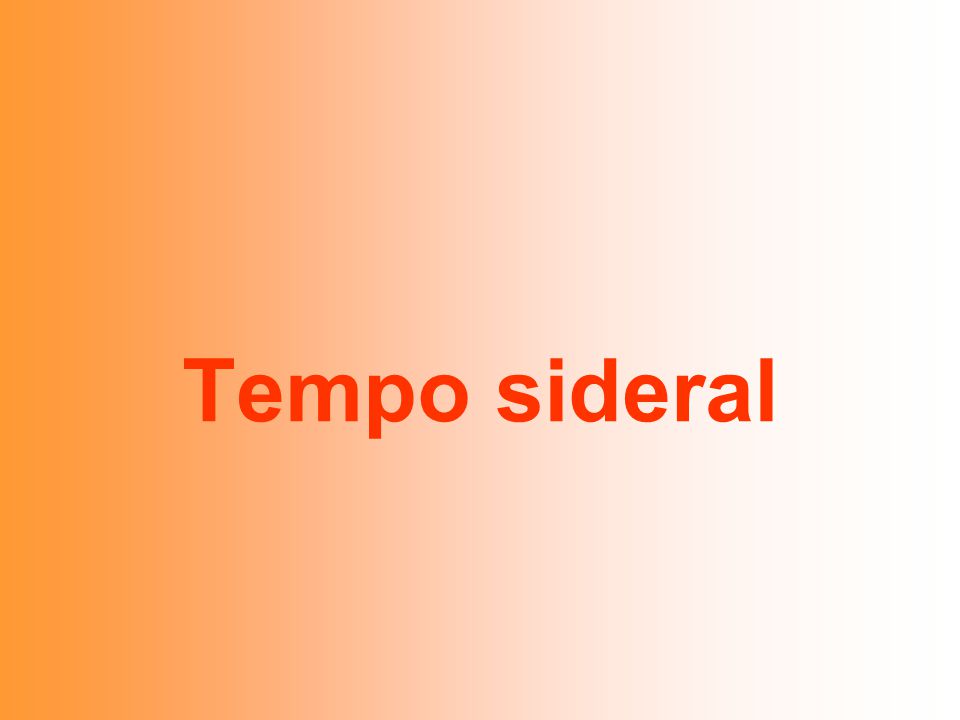The image features a landscape-oriented, gradient background that transitions from dark orange on the left to white on the right. Centered slightly below the middle are the words "TEMPO SIDERAL" in a bold, dark red sans serif font. The text stands out prominently against the smooth, seamless transition of the background colors, making it a striking yet simple graphic design. The font style is straightforward and unembellished, emphasizing clarity and readability.